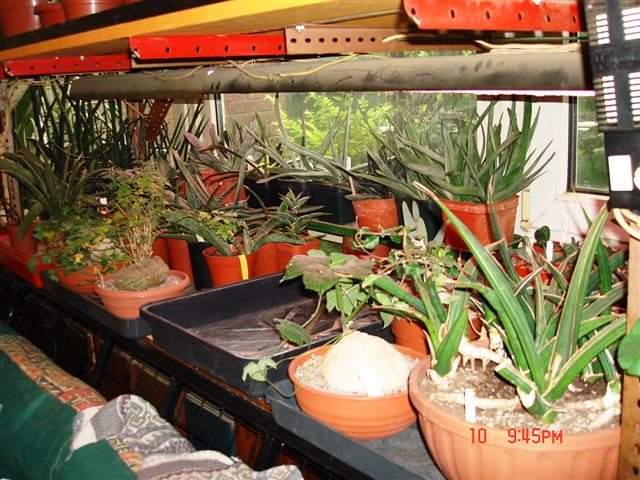This image captures the interior of a modest greenhouse, possibly part of a pottery shop, taken at 9.45 PM in October, as indicated by a timestamp in the bottom right corner. The greenhouse houses an abundance of potted plants, predominantly succulents, which are planted in reddish-brown clay pots neatly organized in black trays. These trays are placed on two large, utilitarian shelves supported by bright red metallic beams. The shelves, while functional, appear hastily assembled. A window in the background offers a view of more plants and a brick wall outside. The scene is illuminated by the camera's flash, casting distinct shadows from the plants' leaves, enhancing the detailed texture of the foliage.